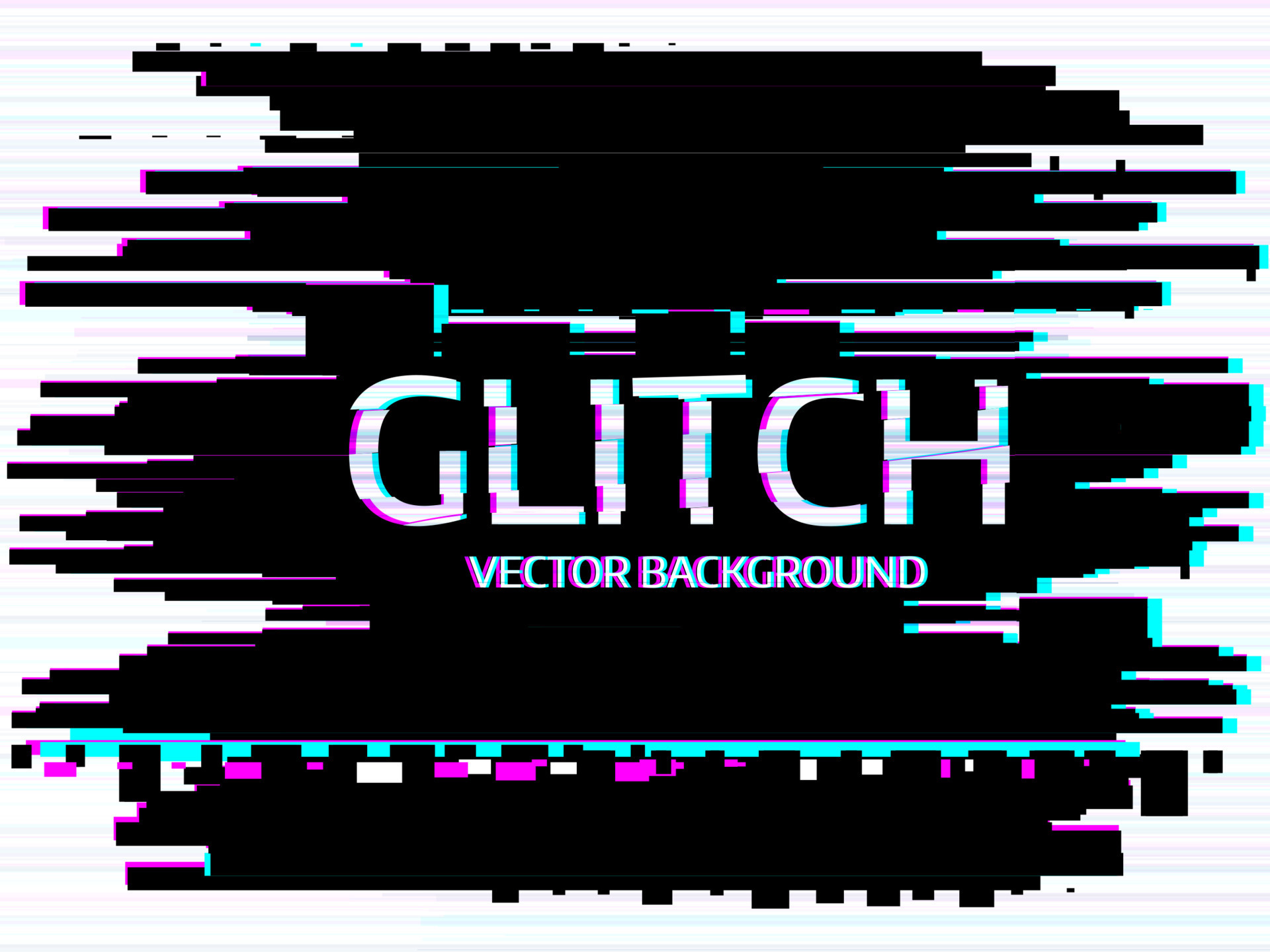The image is digital art presented in a rectangular, landscape orientation. The primary focus is the text "GLITCH" in large, all-caps white letters, centrally positioned. Below "GLITCH," in smaller yet still capitalized letters, is the phrase "VECTOR BACKGROUND." The background is a mix of white, purple, and blue horizontal lines, creating a repetitive pattern that gives the illusion of movement. Surrounding these lines is a blotchy, digitized black area with missing sections in the center and towards the bottom, revealing the colorful lines beneath. The horizontal lines exhibit gradients with aqua blue on the lower right and pink on the upper left, enhancing the pixelated, retro aesthetic. The black area does not extend fully to the top, bottom, or sides of the image, leaving portions of the lines visible at these edges, adding to the image's fragmented, glitchy effect. The intricate detailing and color scheme contribute to a highly stylized, pixel art visual.